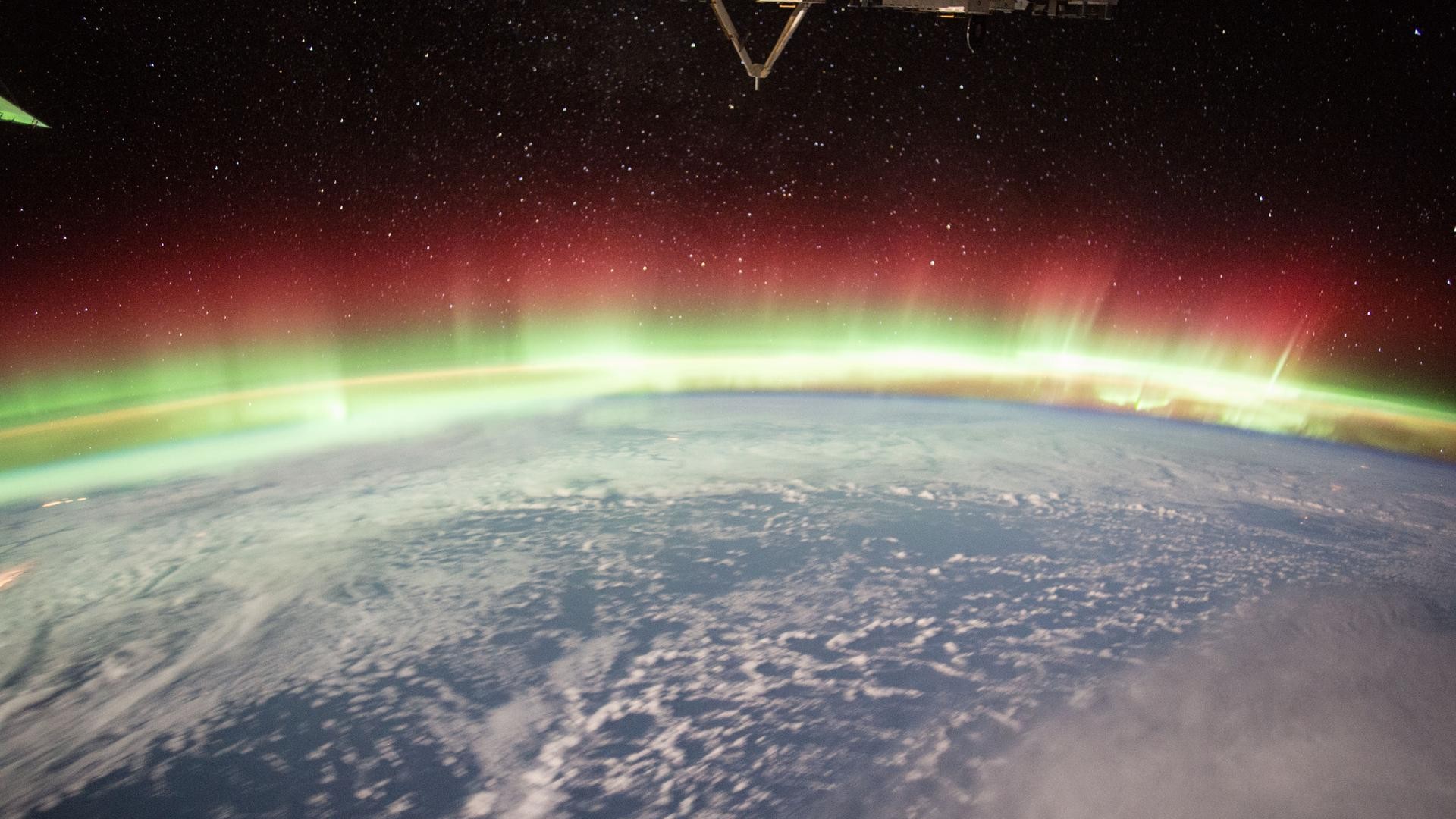This image captures a breathtaking view of Earth from space, emphasizing the planet's curvature and the striking visual phenomena surrounding it. The lower portion of the photograph showcases the vibrant blue surface of Earth, adorned with dynamic cloud patterns and hints of gray. Above this, an ethereal glow emerges, seemingly depicting the Aurora Borealis, with hues transitioning from greenish-yellow closer to the surface to vibrant reddish-pink extending further out. This mesmerizing aura wraps around the circumference of the Earth and creates a misty, fog-like effect. The vast expanse of space frames the spectacle, outlined with a black sky dotted with countless white stars. Adding to the composition, a metallic V-shaped object, likely part of a spacecraft such as the International Space Station, hovers at the upper portion of the image. Additionally, the top left corner features a faint green object, resembling a blade of grass but presumably part of the atmospheric phenomena. The overall vibe is both awe-inspiring and slightly ominous, capturing the mysterious beauty and complexity of our planet from the stunning vantage point of space.